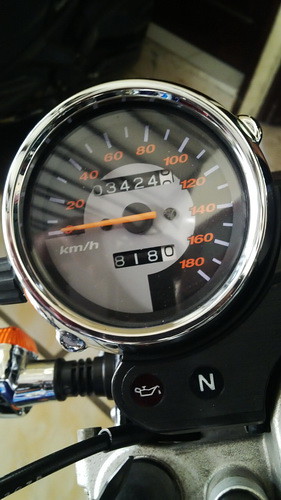Here is a detailed, descriptive caption based on the provided description:

---

The photograph features a close-up view of a gauge set against a predominantly dark background. In the immediate forefront, the primary focus is on a meticulously detailed gauge assembly. At the bottom of the image, there is a gray pipe extending horizontally, affixed to the wall, with two circular components attached to it. The first circle, located towards the lower right, is partially obscured with black. The second circle is distinctly black.

Above this pipe setup, there is another black component capped with white, adorned with a minor icon. Emanating from this section is a black hose that connects to yet another black component marked with multiple circle patterns. 

Dominating the center of the image is the main gauge, bordered by a silver circular frame. The face of the gauge is black, featuring small white dashes signifying measurement intervals. Bold orange numbers, ranging from 20 to 180, encircle the face. The orange indicator needle is currently pointing to zero. Additionally, the gauge includes a rectangular display with numerals: "34 24" at the top and "81 80" at the bottom.

The background, while mostly dark, reveals a tan box with a gray strip on top, possibly a wood board standing upright. Further back, a brown wooden table is visible, casting shadows of linear elements, with a gray and an orange object faintly perceptible on its surface.